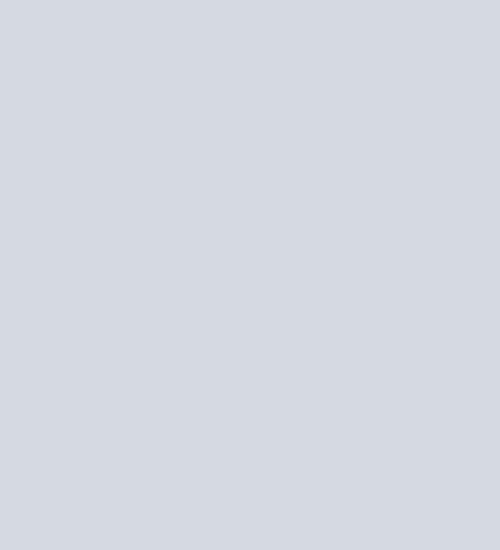The image depicts a blank, light gray rectangle in portrait orientation. The screen is completely devoid of any text, images, or distinguishing features. The entire visual field is uniformly gray, with no discernible variations or elements on either side. It presents a clear, uninterrupted expanse of color, emphasizing its emptiness and simplicity.